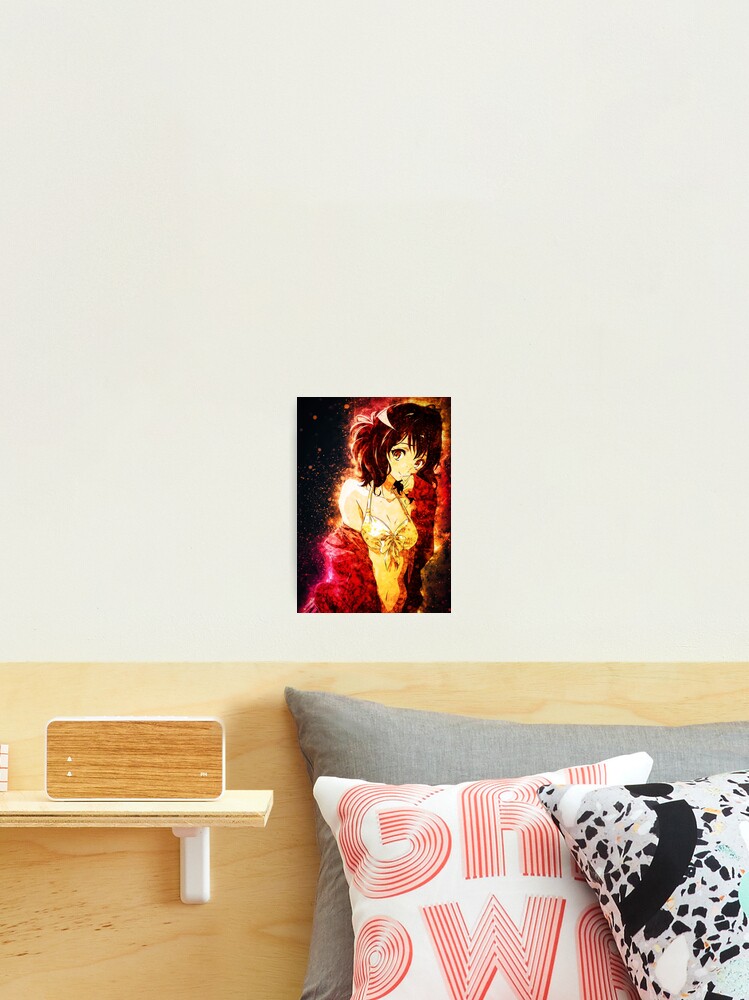In this detailed indoor photograph, we see a cozy arrangement featuring a light brown wooden panel at the bottom. On the bottom right corner of the paneling, three pillows are evident: the first in the back is a long dark gray pillow, the second in the center is a white pillow with red letters that appear to spell "G-R-I-W" or "G-A-W," and the third is a white pillow with a black and white pattern resembling cheetah print or abstract black triangles. To the left of the wooden paneling, there's a small wooden shelf holding what seems to be a phone with a wooden case.

Above the paneling is a striking unframed poster on a white wall. The poster features an anime girl, likely from the series "The Misfit of Demon King Academy." She has short brown hair, red eyes, and appears to be blushing, with one hand near her mouth. She is dressed in a yellow bikini or bra top, with a red jacket, and a surrounding red and yellow aura. She leans against a wall that is depicted on her right side.